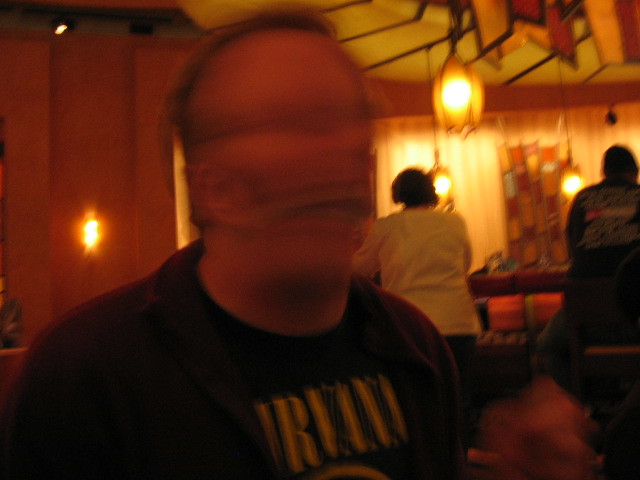In a warmly lit indoor setting, likely a restaurant or bar, a man is prominently featured at the center of the image. His face is heavily blurred due to motion, appearing distorted with an elongated mouth and visible but indistinct teeth. He wears glasses, has a receding hairline, and black hair. The man is dressed in a black T-shirt with yellow "Nirvana" text and a burgundy jacket over it. Surrounding him, the ambiance showcases unique decor, including hanging lights that resemble unbloomed flowers, casting a yellow or orange glow. The ceiling and walls feature colorful, translucent tiles arranged in both square and rectangular patterns. In the background, two other individuals are seated at the bar on stools; one is a woman in a white blouse with short to medium length hair, and the other is a man in a black T-shirt with white writing. The entire scene is bathed in natural lighting, contributing to the image's warm and inviting atmosphere.